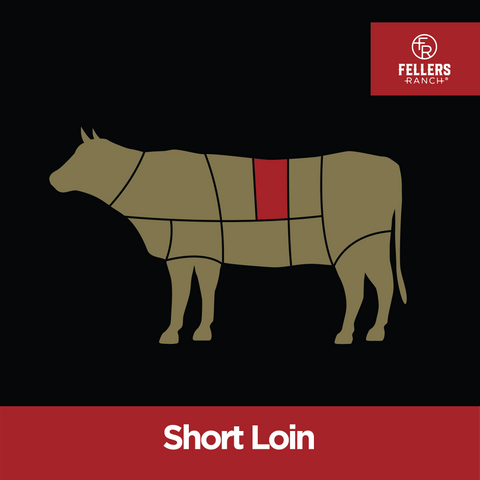The image is a computer-generated graphic featuring a tan cow with outlined sections against a black background. The cow, which faces left, has detailed delineations showing various meat cuts, with approximately 14 different sections identified by black lines. Prominently, a vertical rectangular section on the cow's back is highlighted in red, indicating the "short loin." The cow has two horns, four legs, a tail, and hooves, but lacks facial details. In the upper right corner, a red box contains a circular logo with the letters "FR" in white and the words "Feller's Ranch" in white, all caps, beneath it. At the bottom of the image, a red horizontal rectangle features the words "short loin" in white.